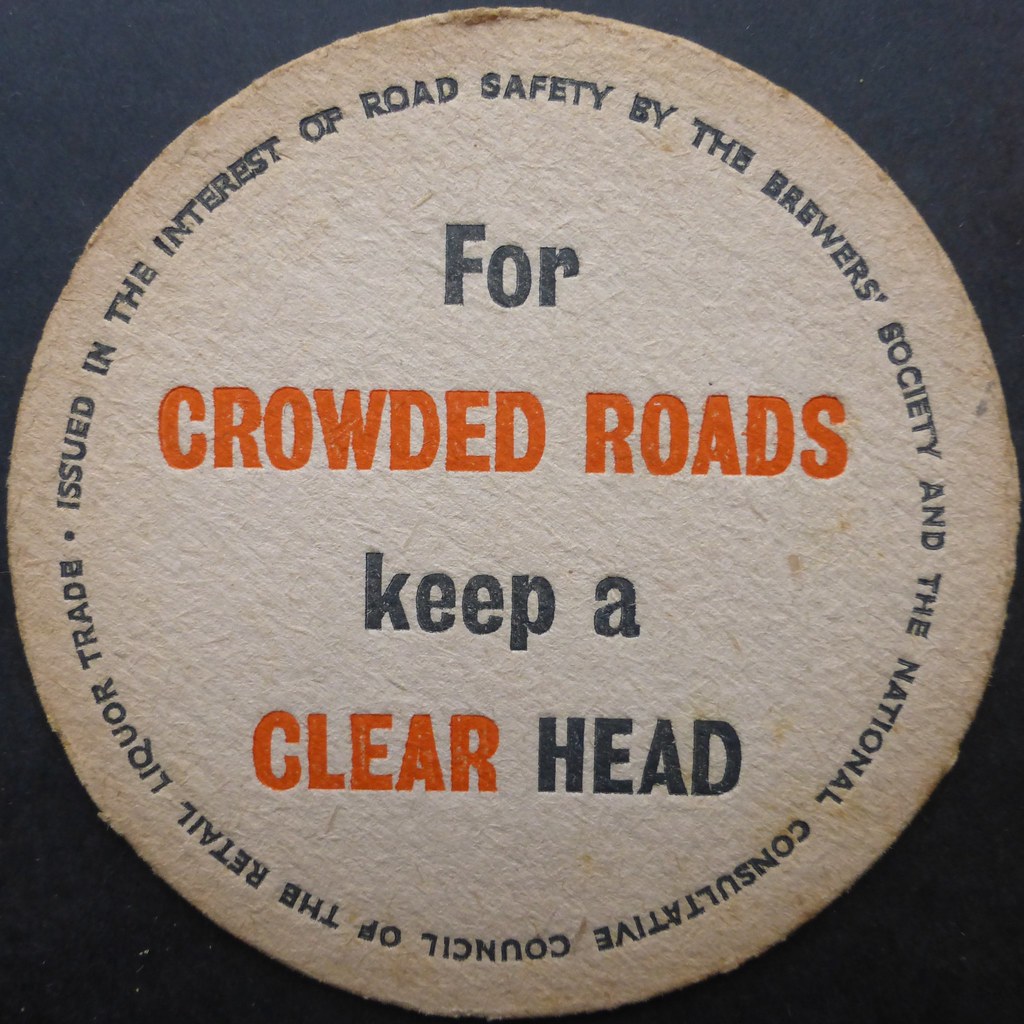This photograph features a single, centrally positioned circular object on a solid, dark-colored background, which could be navy blue or black. The object itself is a tan-colored circle, which appears to be either a coaster or a fabric patch. The materials suggest it may be made of felt or similar fabric. The circular object prominently displays a message in blue and orange text reading, "For crowded roads, keep a clear head." Surrounding this central proclamation, written in blue text, is an inscription that reads, "Issued in the interest of road safety by the Brewer Society and the National Consultative Council of the Retail Liquor Trade." The detailed design and clear, central positioning focus the viewer's attention entirely on this object, emphasizing its potential purpose related to promoting road safety.